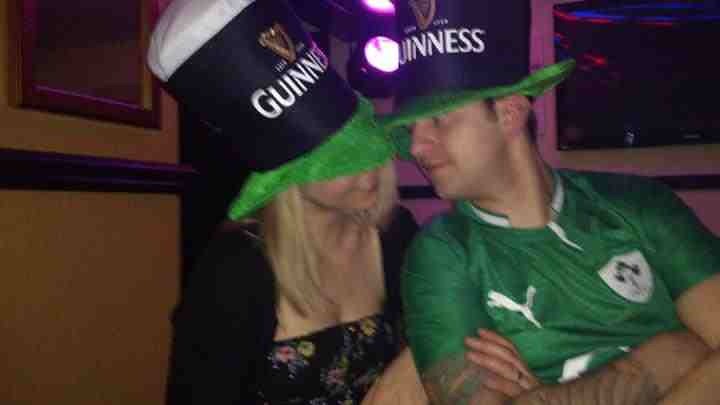In an indoor bar setting with a festive atmosphere, a blonde woman and a white man pose for a photograph. The woman is dressed in a low-cut black dress adorned with flowers and a matching black sweater, her hair cascading just past her shoulders. She clings to the arm of the man beside her. He wears a green polo shirt featuring the Puma logo on the left side and a shield logo on the right side, with a hint of white on the collar. Both are sporting oversized Guinness hats with green brims, showcasing the iconic harp logo. The man stands with his arms crossed, leaning towards the smiling woman who gazes up at him. Behind them, a tan wall with a decorative wooden piece and a pink-framed window can be seen, adding to the cozy bar ambiance. The couple's close stance and affectionate gestures suggest a moment of shared joy, possibly amidst a celebratory event like St. Patrick's Day.